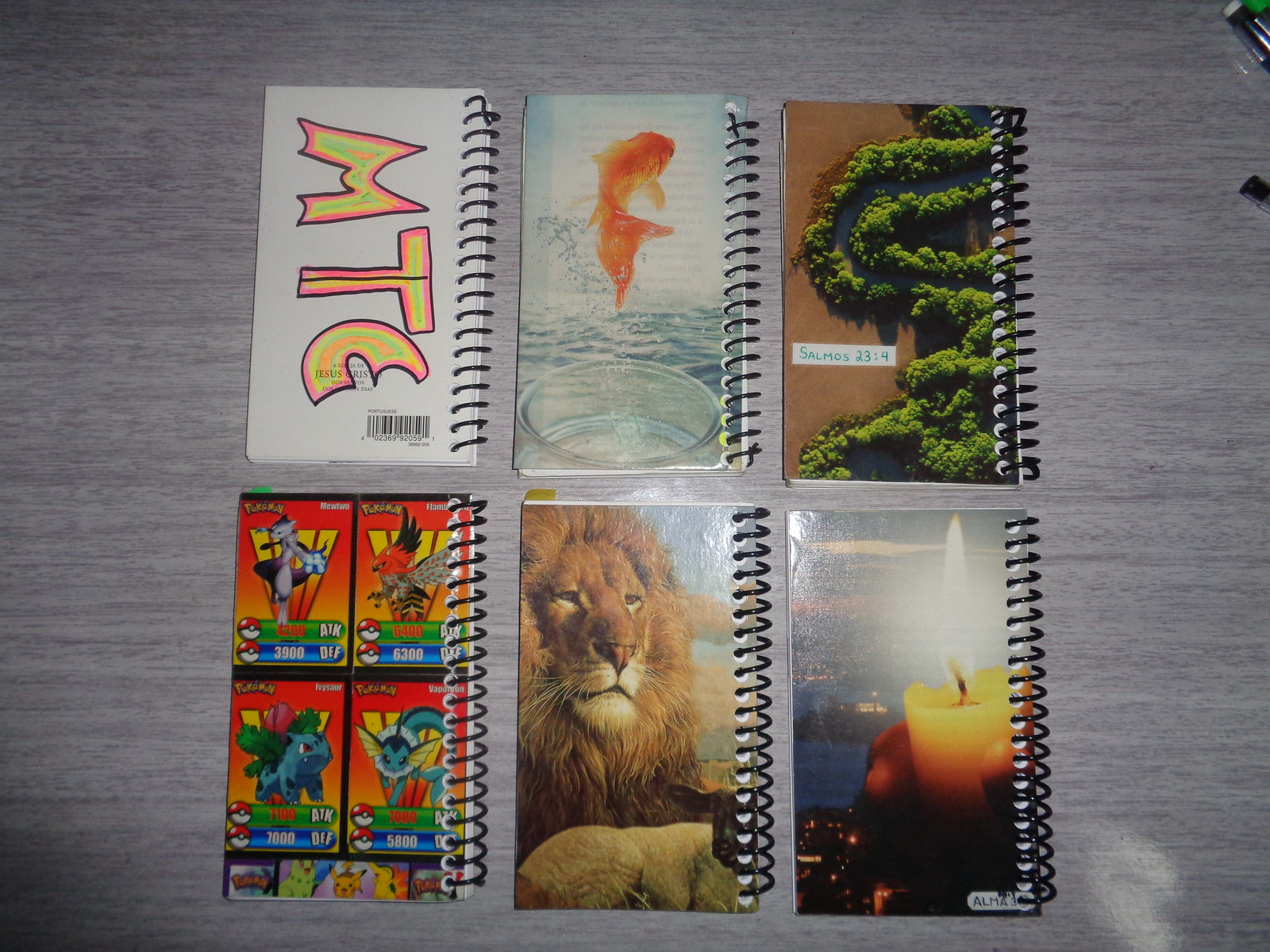This photograph depicts six spiral notebooks arranged in two rows on a gray desk. Each notebook features a distinctive cover design. Starting from the top left, the first notebook showcases the initials "MTC" in a vibrant, colorful, cartoony font. Next to it, on the top middle, there's a depiction of an orange goldfish leaping from its bowl, with a watery background. The top right notebook displays the text "Salmos 23:4" set against a scenic backdrop of green trees and a dirt field. 

On the bottom left, one notebook cover features images reminiscent of video game screenshots, including several recognizable Pokemon characters like Mewtwo and Pikachu, against a red and orange background. Beside it, in the bottom middle, another cover presents a majestic lion resting in a desert field. The final notebook, positioned at the bottom right, shows a lit candle with a night cityscape illuminated in the background, featuring reflective water and evening lights.

Overall, this eclectic collection of notebooks is captured from a top-down perspective, highlighting their unique thematic covers on a gray wooden table.